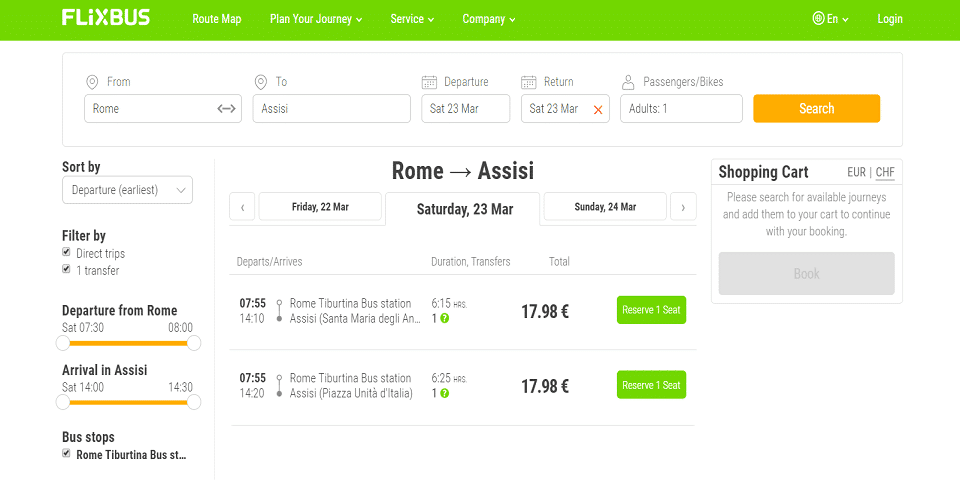The Flixbus website is displayed on a wide desktop screen, characterized by a predominantly white interface with a green top bar. This platform, reminiscent of a government or public transportation site, allows users to book bus rides. The specific itinerary shown is a trip from Rome to Assisi, with departure scheduled for Saturday, March 23rd, and a return on the same day. One adult passenger is selected for this journey. The page presents two different bus options for the departure, with one taking 10 minutes longer than the other. Both options currently have availability. Filters and adjustment settings are visible on the left side of the screen, providing standard customization options for the search results.